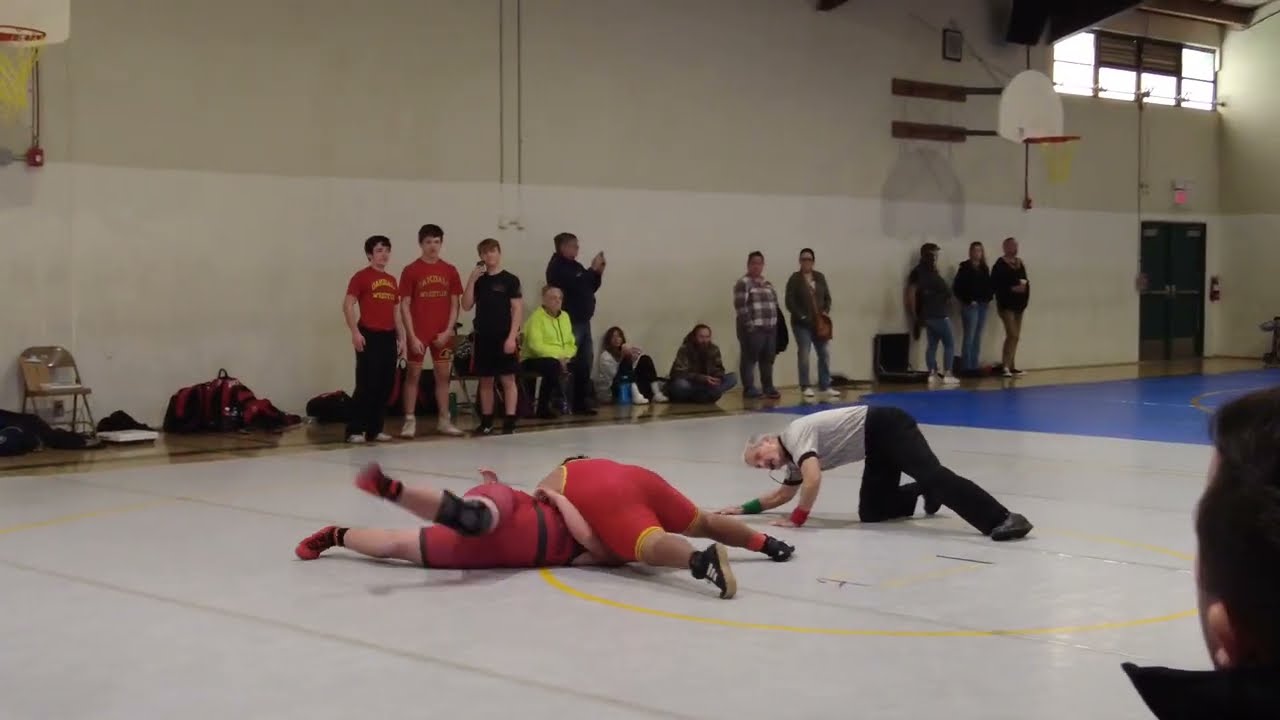This detailed color photograph showcases an amateur wrestling match set in a high school gymnasium with gray and white walls—the upper half in gray and the lower half in white. The focal point is a gray wrestling mat with a yellow circle at its center, contrasted by a blue mat in the background. Two wrestlers, both in red singlets, are in a tense moment of the match. One wrestler is pinning the other to the mat, with the pinned wrestler attempting to escape by lifting his right hip and rolling over to avoid the pin. Positioned closely, a referee with gray hair, dressed in a white shirt and black pants, is kneeling down to closely monitor the wrestlers' shoulder positions. Scattered around the wrestling area are various gym bags and spectators, some of whom are family members, identifiable by their casual attire and action of capturing moments on cell phones. In addition to the sporting action, there are elements typical of a gym setting such as a basketball hoop and a window in the far right corner that lets light into the facility. The photograph, taken in landscape orientation, captures the intense and dynamic nature of the wrestling match while providing a clear view of the bustling gym atmosphere.